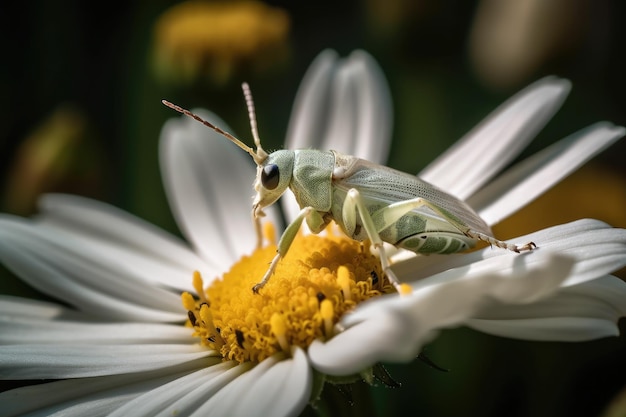In the center of the image, a pristine white daisy with delicate petals surrounds a circular, vibrant yellow core, which is rich with pollen. Perched on the yellow center is a small, greenish-white insect, resembling a grasshopper, with its body partially blending into the petals. The bug has distinct features: two antennas forming a V shape, a large black eye, and legs marked with a mix of light and dark green patterns. Notably, one of its legs has yellow pollen dusted on it, suggesting its active role in pollination. The background of the image is artistically blurred, highlighting the daisy and bug while offering hints of other plants and flowers in shades of green, yellow, and white. This horizontal, rectangular photograph captures a moment of nature’s intricate beauty and the symbiotic relationships that sustain it.